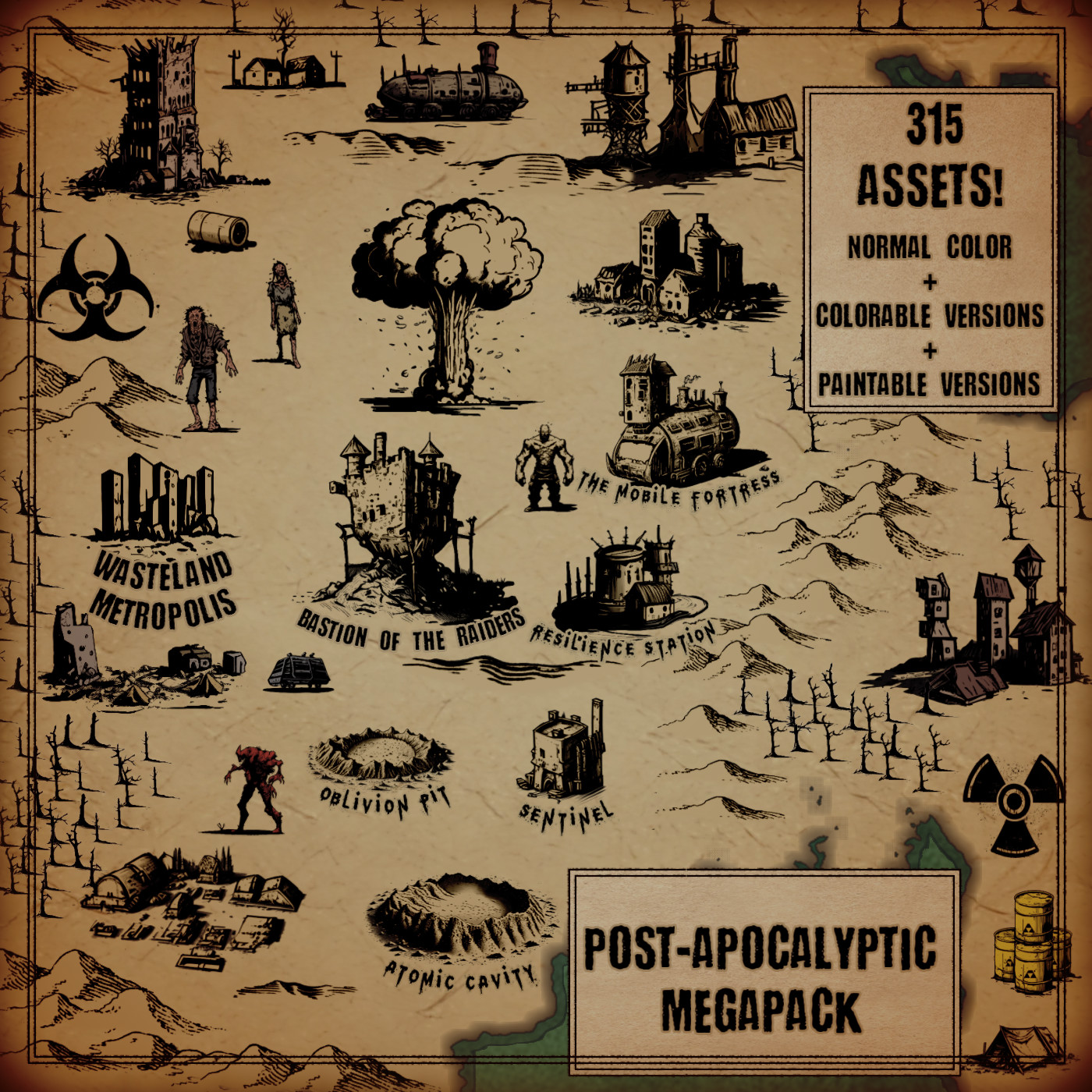This image is a highly detailed poster promoting a "Post-Apocalyptic Mega Pack" for a game, featuring 315 assets available in normal colors, colorable versions, and paintable versions. The overall aesthetics mimic a post-apocalyptic wasteland, characterized by a burnt, smoky look that accentuates the desolate atmosphere. The top left showcases broken-down buildings and a wasteland landscape, dotted with ominous mushroom clouds. Key locations within this pack include the Wasteland Metropolis, a sprawling urban ruin; Bastion of the Raiders, resembling a large medieval castle; the Mobile Fortress, an imposing truck with a house structure on its top; and the Resilience Station. Additional notable sites are the Oblivion Pit, a foreboding deep pit; the Sentinel, a small, castle-like structure; and the Atomic Cavity, a large, crater-like formation. Characters, including red creatures, zombie-like beings, and a large figure near the Mobile Fortress, further enrich the thematic setting. A radioactive sign located at the bottom right, alongside the comprehensive list of assets, encapsulates the pack's grim and gritty motif, ideal for game map construction or storytelling.